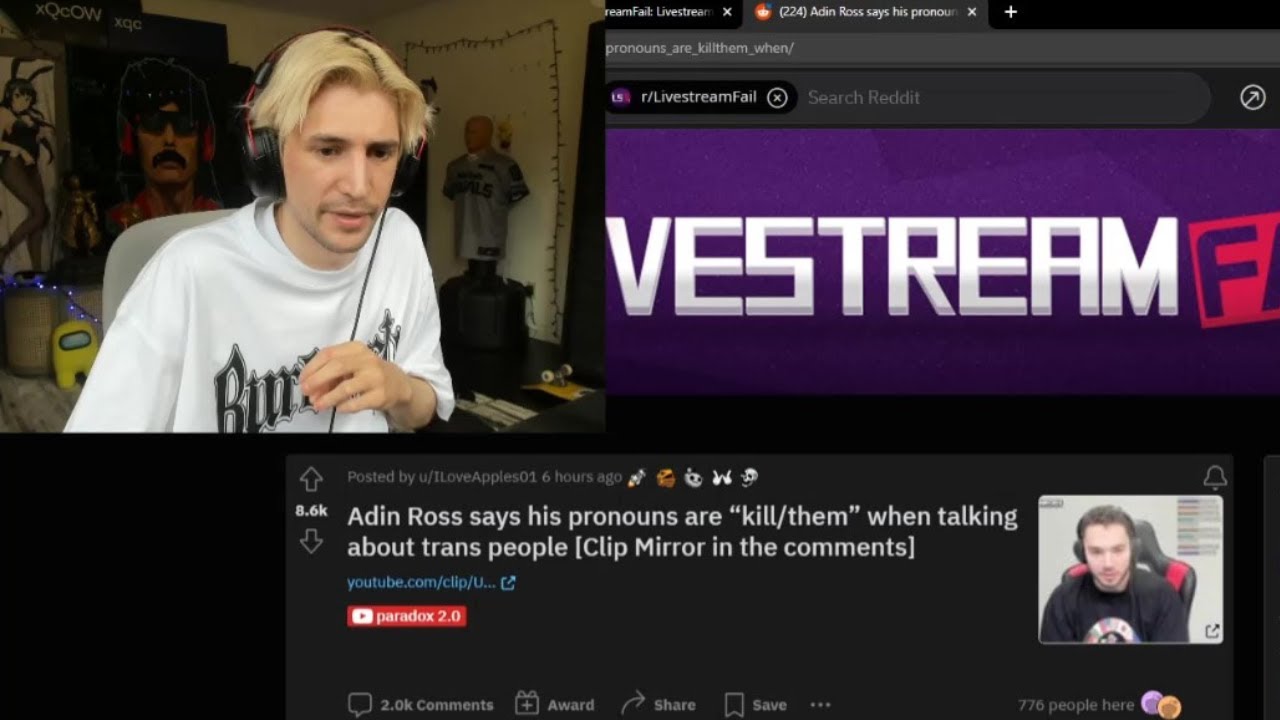The image showcases a webpage with a distinct purple-themed interface. The central focus is a logo reading "V-E-S-T-R-E-A-M" in white, 3D-styled letters with light purple outlines against a dark purple background. Adjacent to the logo, a red banner with partially cut-off dark purple letters—an "F" and part of another letter—is visible. Above this, at the top center of the image, a faintly visible phrase includes "live stream" followed by an "X".

Midway down the image, a black search bar with a white plus sign is seen, followed by a dark gray search bar containing the phrase "pronouns - R - kill K-I-L-L-T-H-E-M - when, killing them when /".

A black banner underneath reads "R / live stream fail" with a small circle and an "X" inside it. Below this, a dark gray banner features the text "search Reddit".

To the left of the "V-E-S-T-R-E-A-M" logo, there's an image of a man in his 20s or 30s with parted, straight blonde hair, wearing black headphones and a white t-shirt with black writing. He is seated in a desk chair, partly cut off at the waist, with posters covering the wall behind him and a headphone cord visible.

At the bottom of the image, a banner states: "Aden Ross says his pronouns are kill / them when talking about trans people". This is followed by a clickable link "clip here in the comments", and another section noting the post by "u / I love apples 01" from six hours ago, accompanied by five tiny emojis and an upvote count of 8.6k.

Further down, the text under "Aden Ross says his pronouns…" includes a blue YouTube link and a red banner marked "Paradox 2.0", indicating a playable video.

On the lower right, a small image of another individual with headphones and a black shirt in his 20s or 30s is seen. Beneath this, it shows "2.0k comments" with options to gift, share, and save the post, followed by three dots. Finally, at the bottom right corner, it indicates that "776 people are here".